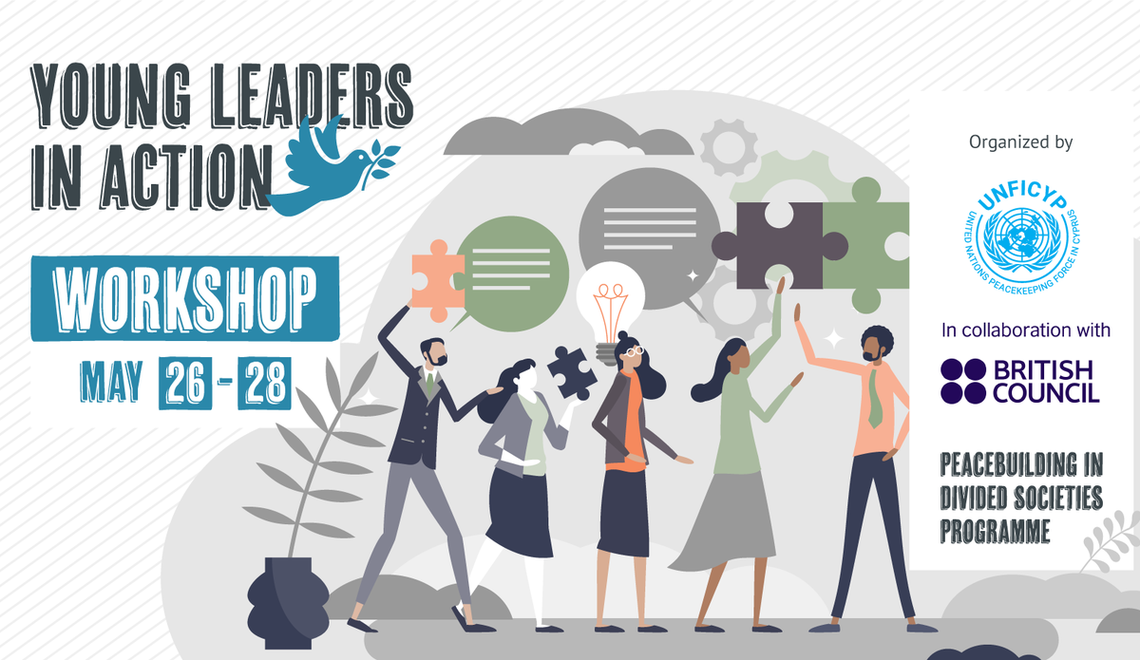The poster advertises a "Young Leaders in Action" workshop scheduled for May 26th to 28th. At the top left, the title is prominently displayed in black, alongside a logo featuring a blue dove holding an olive branch, symbolizing peace. Directly beneath this, "WORKSHOP" is clearly written in white text on a blue rectangle, with the dates below it in blue. 

The central part of the poster showcases an illustration of five diverse individuals under a gray sky with muted clouds and a faint sun. Each person is interacting with large puzzle pieces in shades of orange, blue, dark gray, and light green. The first person, a man in a suit, holds an orange puzzle piece overhead, with green text emerging from his mouth. To his right, a woman holds a blue puzzle piece, and further right, two individuals hold gray and green puzzle pieces that are connected. Their surroundings include a black planter with a gray frond leaf, as well as various other flora and abstract shapes like cogwheels and a light bulb.

On the right side of the poster, a white vertical banner indicates that the event is organized by UNFICYP (United Nations Peacekeeping Force in Cyprus) in collaboration with the British Council Peacebuilding and Divided Societies Program. The banner includes a circular arrangement of text around a globe logo and features the British Council's four-circle logo alongside decorative elements. The overall color scheme combines navy blue, gray, muted green, peachy orange, and black.